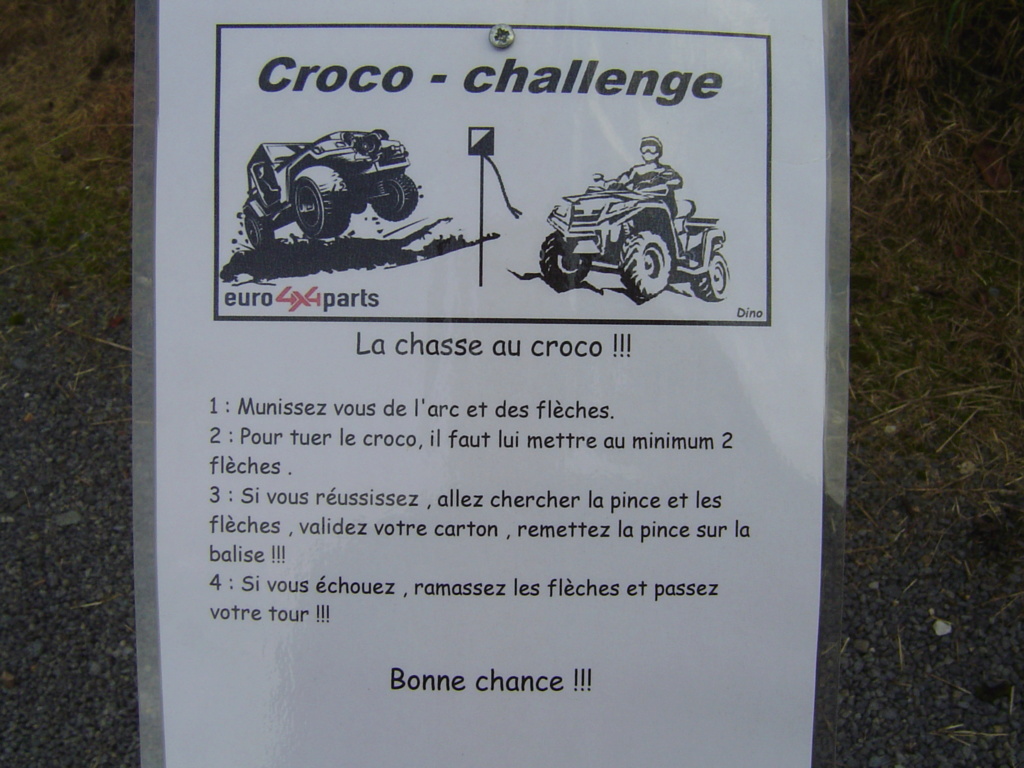The image depicts a laminated flyer, approximately 8.5x11 inches, affixed to an unseen surface with a silver screw through the top center. The flyer, set against a dark ground background covered with dirt, twigs, and grass, is protected by a clear plastic covering showing the edges. The flyer features a black-outlined rectangle at the top, labeled "Kroko Challenge," with two black and white outlined images: a jeep driving over what looks like a silhouetted map of Long Island on the left, and a person with large sunglasses on a four-wheel ATV perched on a rocky crag on the right. "Euro 4x4 Parts" is prominently listed below the images, with "4x4" in red font. The centerpiece of the flyer is the bold text "La Chasse au Kroko!!!," followed by four left-aligned numbered bullet points in Comic Sans font containing rules or guidelines in French. Centered at the bottom, the phrase "Bonne Chance!!!" concludes the text. The entire flyer, including text and images, is in black and white except for the red "4x4."